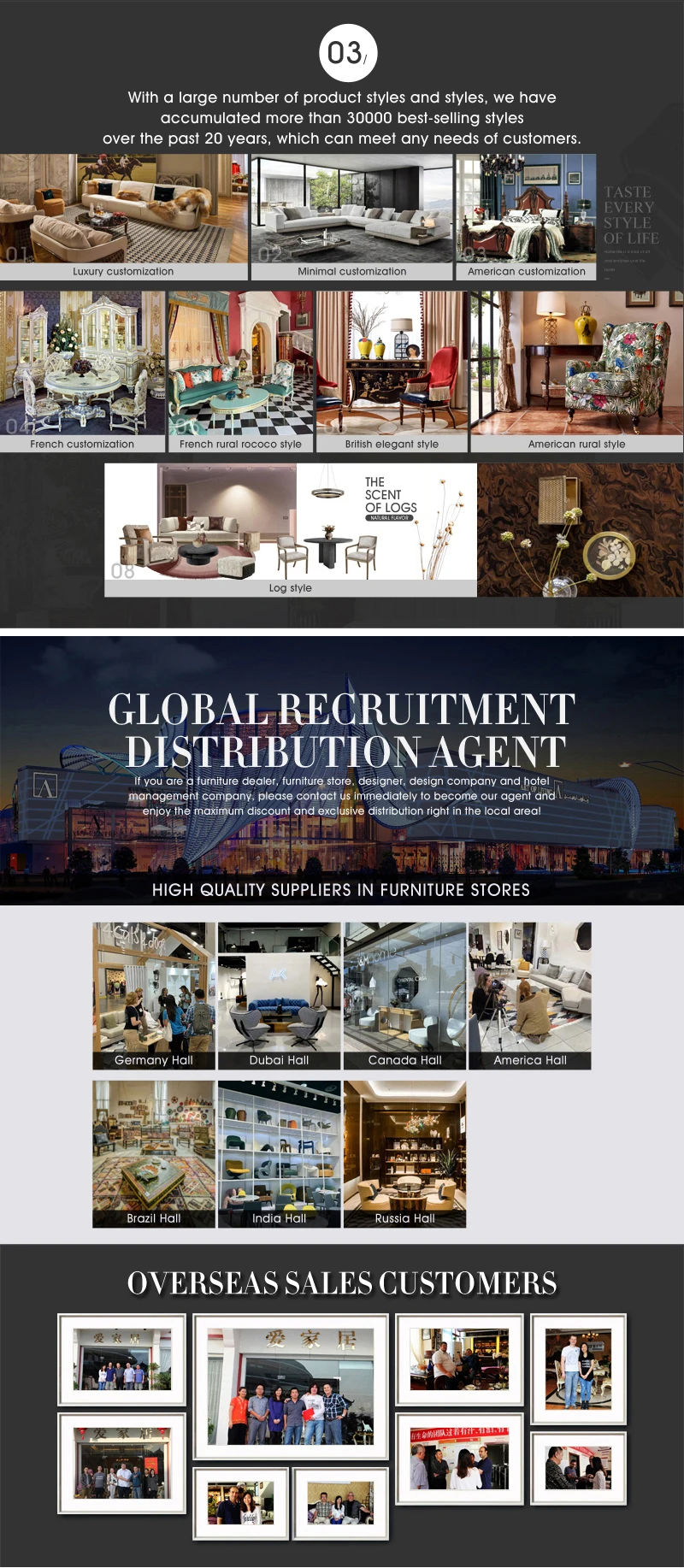This image captures a visually diverse and detailed webpage showcasing an extensive range of furniture styles. 

At the top of the webpage, a black section features a white circle with the number "03" alongside the text, "I'm white." This introduction speaks to the website's vast collection, stating, "With a large number of product styles, we have accumulated more than 30,000 bestselling styles over the past 20 years, which can meet any needs of customers." Although the font is somewhat challenging to read, the message is clear.

Scrolling down, the first visual section displays two tan couches placed on a black and gray rug, transitioning into a more modern living room setting featuring white couches against a black wall, with a tree enhancing the room's elegance. Adjacent to this, the next image presents a blue wall, a black chandelier, and a cherry-stained bed, complemented by gray font that reads, "taste every style of life."

Further down the page, additional images showcase white French-styled furniture. Another image displays a room with a black and white checkered floor, a teal couch adorned with various pillows, a red chair, and a dark wood table. Following this, there's a vibrant chair highlighted with shades of olive, blue, pink, and orange, positioned with a table in the background.

Continuing to scroll, the page reveals another set of tan furniture accompanied by text stating, "the scent of something," and an announcement for "global recruitment distribution agent," alongside a paragraph explaining the benefits to high-quality suppliers and furniture stores.

In the subsequent section, more images showcase a variety of furniture styles, including gray, tan, and white pieces, with each picture captioned beneath. The final segment highlights "overseas sales customers," presenting an array of photographs of individuals and groups, meticulously mounted on a white background with gray frames.

This descriptive webpage serves as a comprehensive visual catalog, illustrating the company's extensive and varied furniture offerings suitable for diverse tastes and styles.